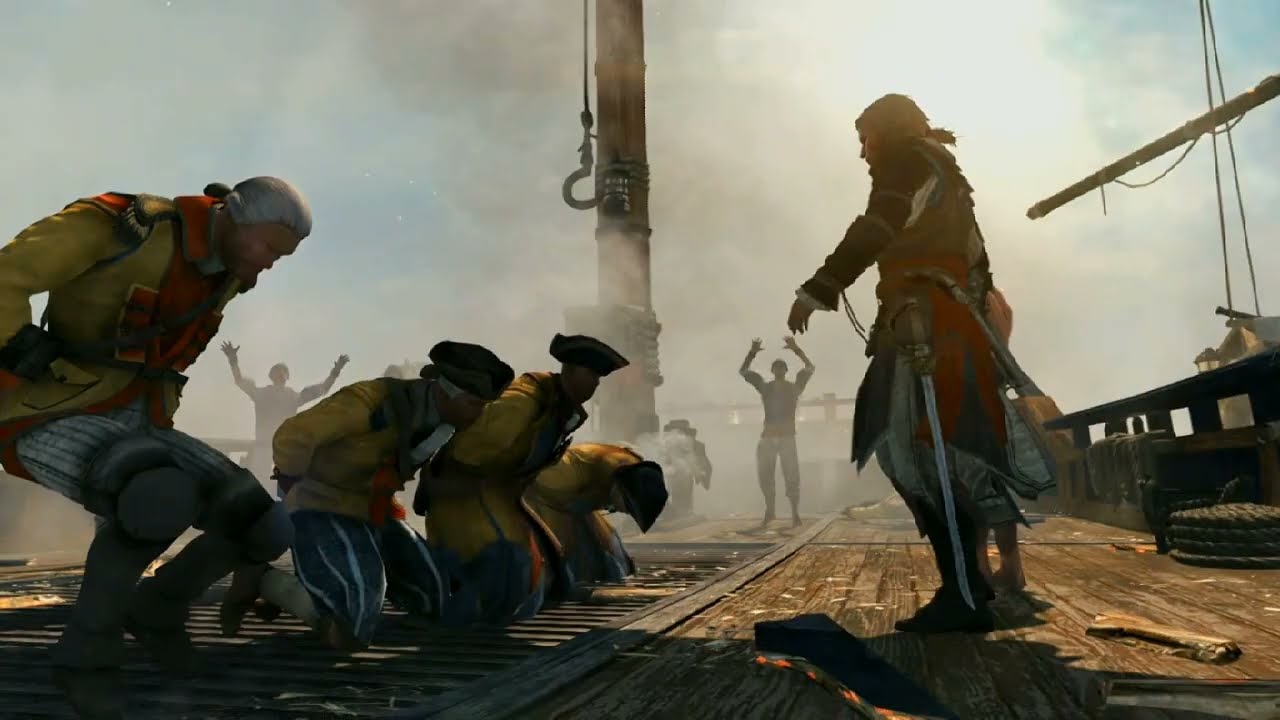In this detailed video game screenshot, the focal point is the deck of a pirate ship captured amidst a tense standoff. In the center of the ship's wooden floor, four men, possibly prisoners or captured sailors, are positioned in various stages of kneeling with their hands tied behind their backs. One of them almost has his head touching the deck, another remains somewhat upright, and one on the far left appears to be in the process of crouching to his knees. To the right, a commanding pirate stands with authority, identifiable by his long black hair tied into a ponytail and a sword sheathed at his side. His gaze is fixed sternly on the kneeling men, suggesting a dire confrontation. The background is filled with dense mist or smoke, hinting at recent combat, probably with gunpowder residue lingering in the air. Behind the central figures, more pirates with their hands raised are visible, further adding to the chaotic atmosphere. Prominent elements of the ship, such as the mast with its pillar and a hanging hook, along with the ship’s boundary fence and a coiled rope, are also distinctly visible against the misty backdrop.